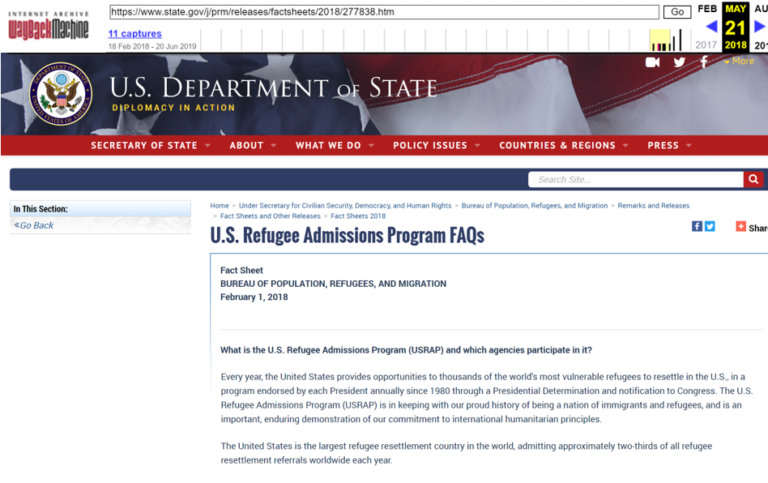This image is a screenshot from the Internet Archive's Wayback Machine. At the top of the screenshot, the address bar is visible, indicating a specific URL. Below the address bar, there is a banner displaying information about the Wayback Machine with the text: "Internet Archive Wayback Machine, 11 captures, 18 February 2018 to 20 June 2019." 

Directly beneath this, part of the United States flag is visible, showcasing the blue field with white stars and a glimpse of the red and white stripes. 

Following the flag is a red banner with the text: "Secretary of State," alongside a navigation menu that includes links for "About," "What We Do," "Policy Issues," "Countries and Regions," and "Press."

Beneath this, a blue banner contains a search box with the prompt "Search site."

Further down, another section labeled "In this section" is visible with an option to "Go back." It introduces the "U.S. Refugee Admissions Program" (FAQ) under the heading "Fact Sheet, Bureau of Population, Refugees and Migration, February 1, 2018."

The text then poses the question, "What is the U.S. Refugee Admissions Program and what agencies participate in it?" followed by a detailed paragraph explaining the program and the involved agencies.